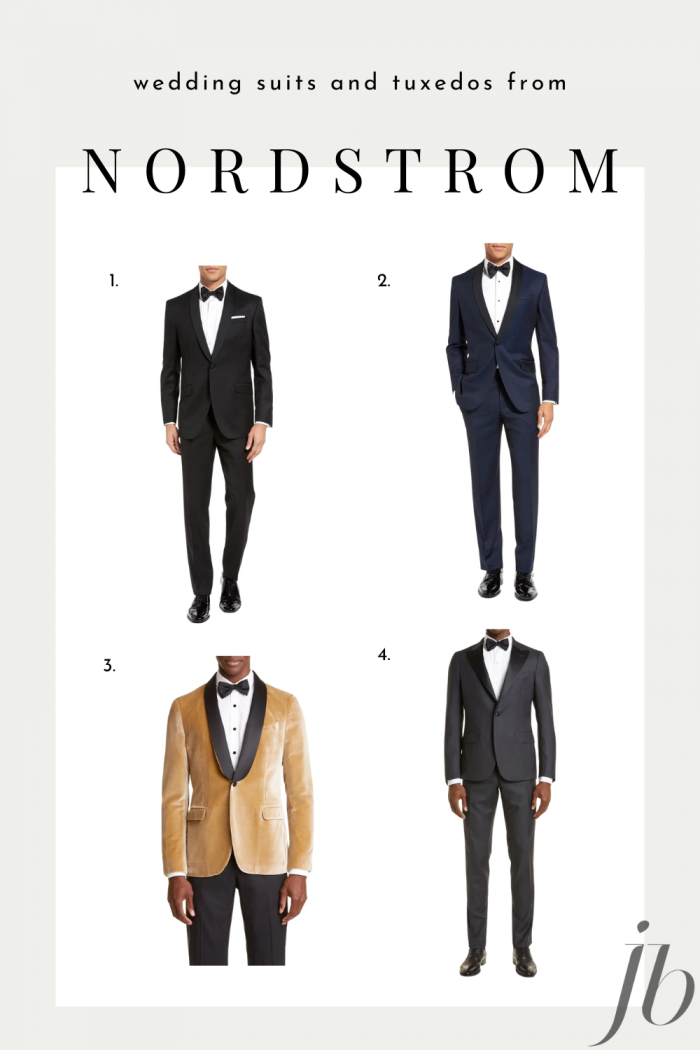The image is an advertisement for wedding suits and tuxedos from Nordstrom, featuring a poster with a prominently displayed gray top border and thinner gray borders around the white central space. The top border, thicker than the rest, contains the text "Wedding Suits and Tuxedos" in small black font, and the word "Nordstrom" slightly bisected at the bottom edge of the border, appearing half in the gray area and half in the white. Below this, the white space showcases four numbered figures, each labeled 1 through 4 at the top left of their respective images.

Number 1, positioned in the top left corner, features a man wearing a black tuxedo with a white shirt and a black bowtie; he is cropped above the mouth. Number 2, seated in the top right corner, displays a man in a navy blue tuxedo with a black bowtie, his right hand placed in his right pocket while his left hand dangles by his side, also cropped just above the mouth. Number 3, located in the bottom left corner, shows a man in a tan or golden jacket with a black outline, black trousers, a white shirt, and a black bowtie, cropped above the mouth as well. Number 4, in the bottom right corner, presents a man in a lighter shade of gray tuxedo with a white shirt and a black bowtie, cropped above the chin. The bottom right corner of the poster features the initials “JB” in a darker gray tone. Each tuxedo is accompanied by black shoes.